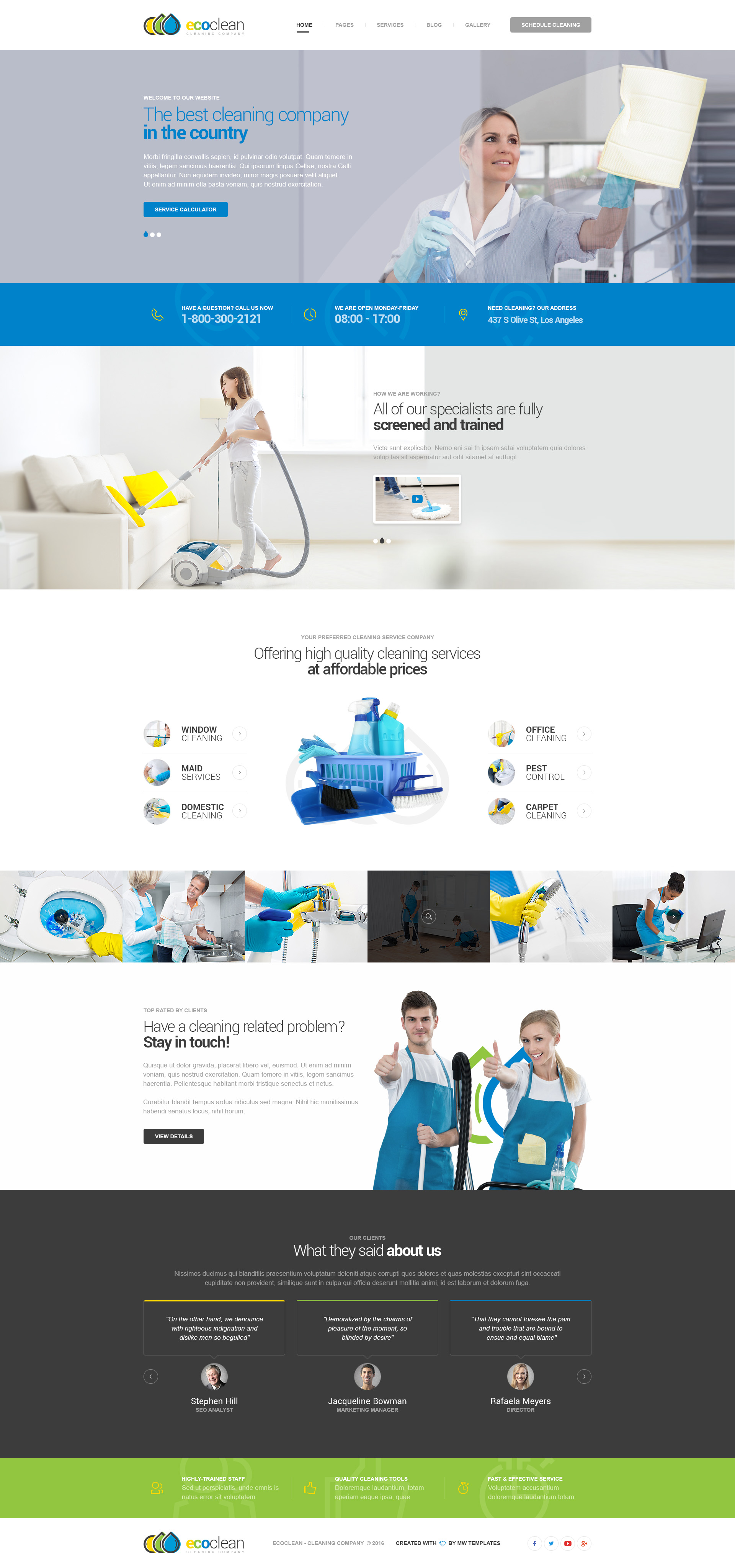The website for the cleaning company features a detailed, eco-friendly theme. Centralized towards the left are two icons resembling rain droplets: the first is medium blue with a black outline, and the second is green with a black outline and two black dashes in its center. Behind these, there's a circular yellow icon with a black border. Adjacent to the icons, the text "Eco Clean" is prominently displayed. "Eco" is written in a gradient transitioning from yellow to medium blue, while "Clean" is in a non-bolded black font.

Below, a streamlined menu appears, though its small size makes the exact options difficult to discern. Beneath this menu, a banner showcases a woman against a gray background, dressed in a traditional maid outfit with a white collared shirt and rolled-up light blue sleeves. Wearing gloves, she is spraying a transparent blue spray bottle and wiping a window or screen with a cloth in her left hand. To the woman's left, in blue non-bold lettering, is the slogan "The Best Cleaning Company," followed by the bold text "In The Country."

Further down, a block of white text is accompanied by a blue rectangle with white writing that reads "Service," though the precise details are difficult to decipher due to the small, non-bold font. A blue bar with white writing provides contact information, including the company's phone number (1-800-300-2121), operating hours (08:00-17:00), and address, which is listed towards the right.

Additionally, an image at the bottom of the page shows a woman vacuuming a beige couch adorned with two yellow pillows on each end.